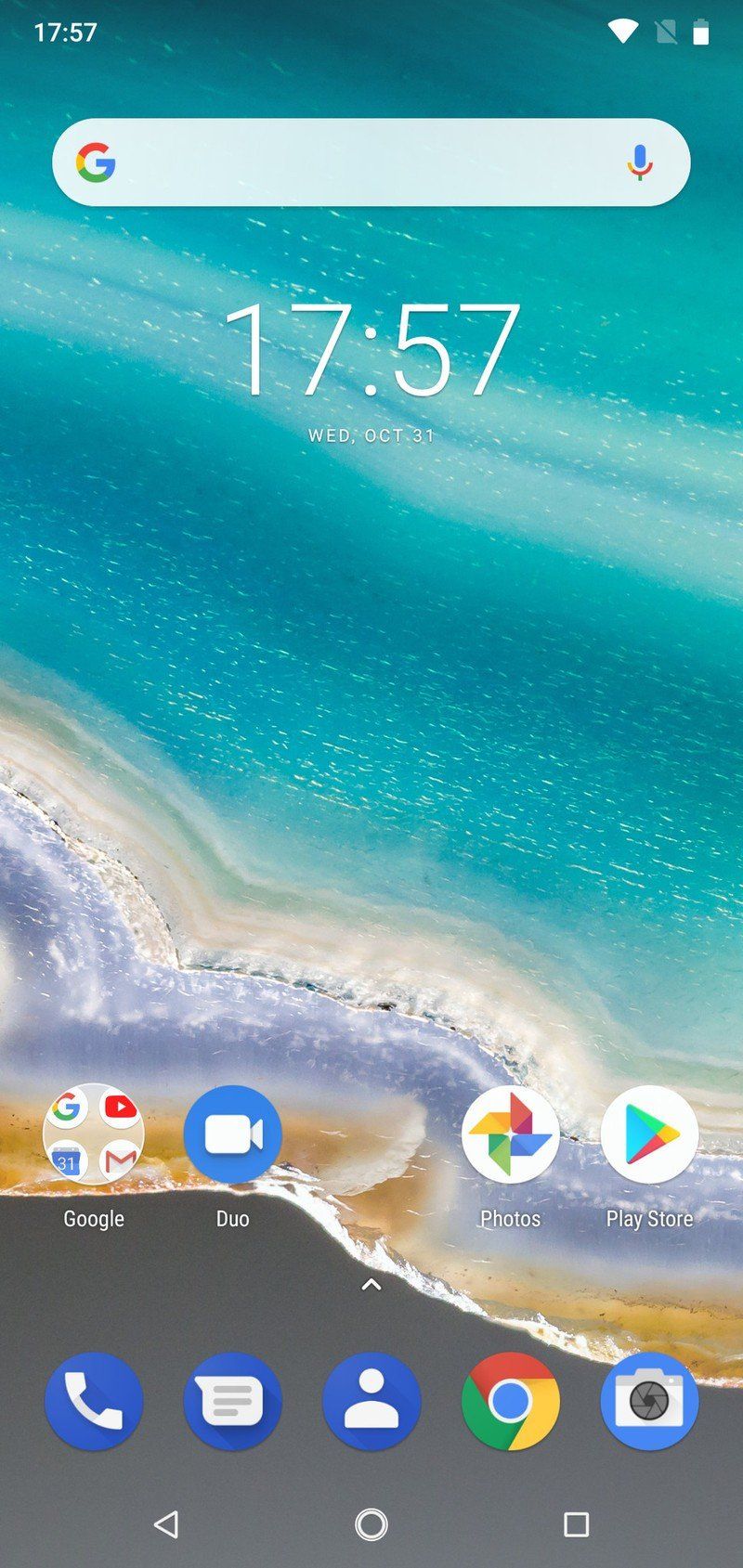A screenshot of a cell phone displays a stunning wallpaper featuring an overhead view of the ocean meeting the sandy shoreline. The top two-thirds of the wallpaper showcases a diagonal shoreline extending from the center-left to the lower-right, with water in mesmerizing shades of aqua green. The sandy shoreline transitions beautifully from tan to white to gray, with visible white caps breaking along the edge. The very bottom of the wallpaper shifts to a steel gray color, adding a stark contrast to the vibrant ocean hues.

At the top-left corner of the screen, "17:57" is displayed in white letters, indicating the current time. On the top-right, icons for the Wi-Fi signal, a battery icon showing about 80% charge, and a square icon with a line through it are aligned. Just beneath this top row, the Google Assistant search bar spans across the screen with the colorful Google "G" on the left and a multicolored microphone icon on the right.

In the center of the screen, "17:57" is prominently shown in large white letters, with "Wednesday, October 31st" written below in smaller white text. At the very bottom, a line of app icons is neatly arranged. The top row includes four icons: a folder for Google Apps, Google Duo, Google Photos, and the Google Play Store. The bottom row starts with three icons featuring solid blue backgrounds. The icons depicted here are a white phone receiver, a text message bubble, and a contacts button. Following these, there is the Google Chrome app icon, capped off by the camera icon also on a blue background.

At the absolute bottom of the screen on the gray background, three navigation icons are displayed in white: a back arrow on the left, a circle in the center, and a square on the right, completing the minimalist yet functional aesthetic of the phone's interface.